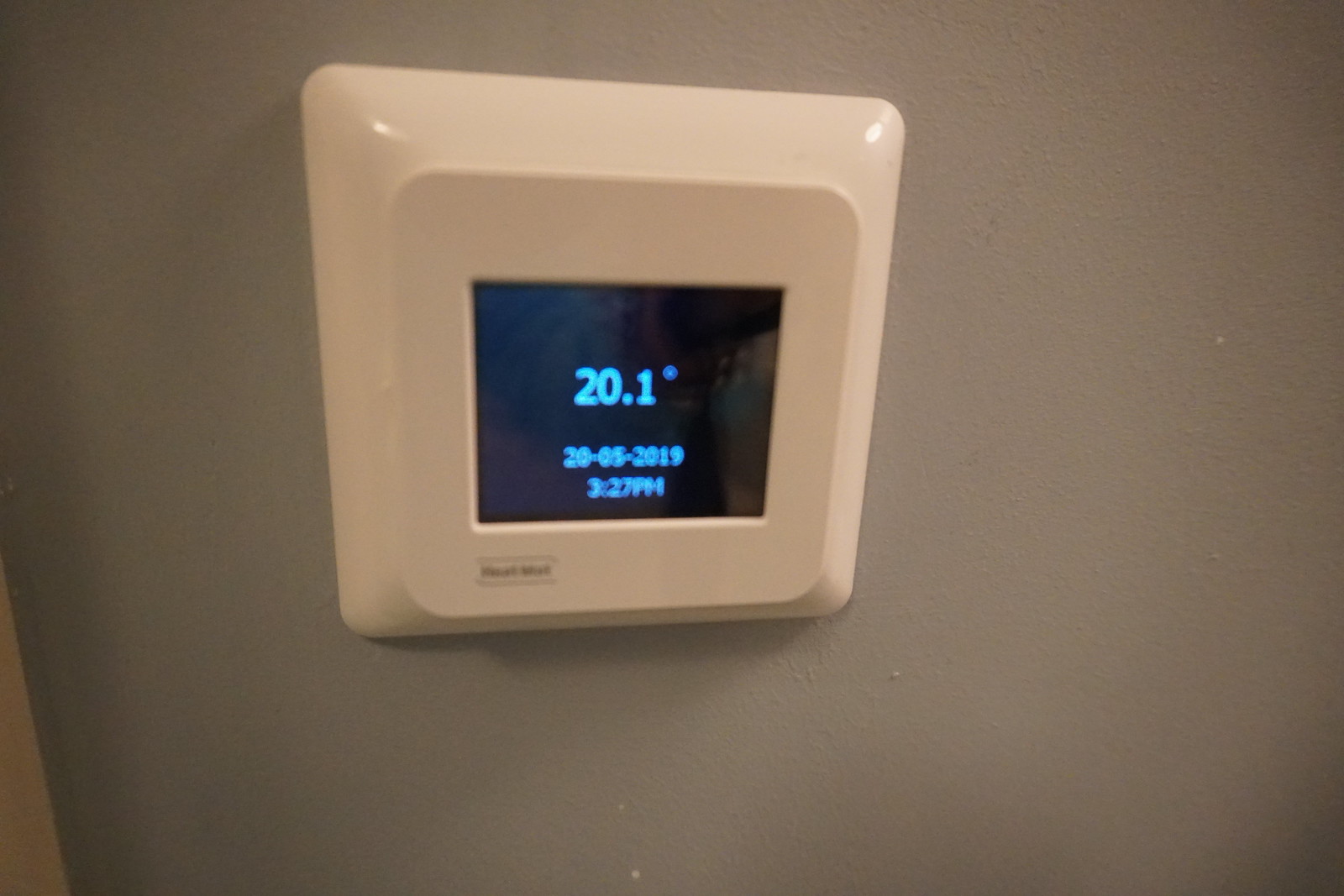This out-of-focus photograph captures a plastic thermostat mounted on a gray, speckled wall. In the lower left corner, there's a hint of a white door frame. The thermostat, which has an indiscernible logo on its bottom left, features a layered square design: a larger square base with a smaller square protruding from it. This smaller square houses a compact LCD or OLED display. Despite the blur, the display shows bright blue text indicating "20.1 degree" at the top. Below this, the date "20-05-2019" is visible, followed by the time "3:27 PM."